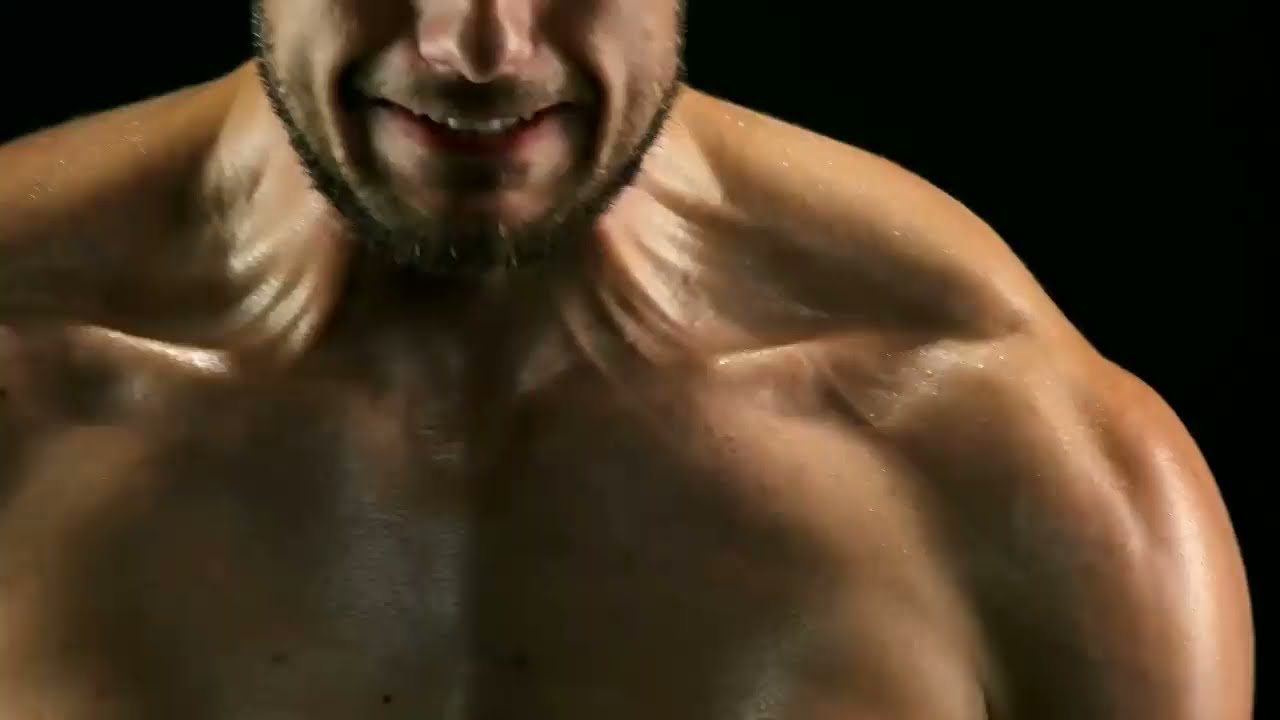The image depicts a close-up shot of a muscular man from just below the eyes to the top of his chest. He appears to be slightly bent forward, flexing his defined pectoral muscles, deltoids, and trapezius. His neck is visibly strained and there's a sheen of sweat on his skin, suggesting exertion. The man has a short beard, slightly longer than stubble, framing his face much like a goatee. He has his mouth slightly open, as if bracing or grunting, conveying an intense effort, possibly similar to the character Wolverine from the X-Men movies. The background is dark, which emphasizes his lean, muscular physique. There aren't many visible veins or striations, but he's evidently very fit with minimal body fat. The image, likely a screenshot from a video or movie, focuses mainly on his upper body strength and strain, capturing the essence of raw physical power.